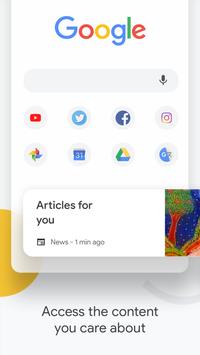The image depicts a vertically oriented screenshot of a Google search page, likely viewed on a mobile phone. The top part of the page is cut off, but prominently displayed in the middle is the iconic Google logo, featuring the letters in blue, red, yellow, and green. Below the logo, there is a stark white search bar, which is slightly different in shade from the background white, and it includes a microphone icon on the right side for voice search.

Below the search bar are two rows of four app icons each. In the first row, from left to right, are YouTube, Twitter, Facebook, and Instagram. The second row includes icons for Google Photos, Calendar, Google Drive, and an unidentified app.

Further down, there is a slightly raised rectangle with the text "Articles for you, news, one minute ago" that introduces a section for personalized articles. To the right of this text, there is a small, illustrative image of a tree against a starry night sky. The sky is blue with white star-like spots, the tree has green leaves and a brown trunk, and there's a reddish tint in the coloration.

The entire content rests on a white background. At the bottom left corner, there is a yellow circle, and to the right, a curved grey line. Centered at the very bottom, there is a message in black text that reads, "Access the content you care about." The top portion of the screen appears to be cut off, but the main focus is maintained on the Google search and associated elements.